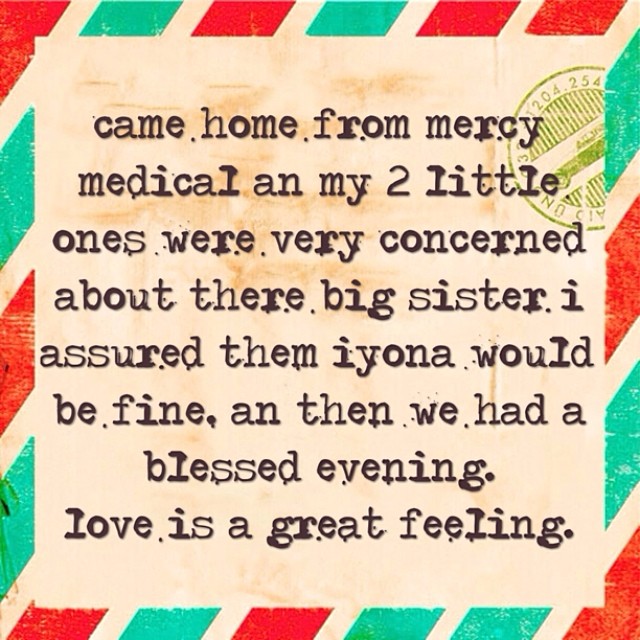This image is designed to resemble a vintage postcard or telegram, complete with red and green dotted borders that alternate and form a frame, revealing a peach-colored background reminiscent of aged paper. At the top right corner, a partially visible green circular stamp features a side profile of a car, along with various numbers and lines, suggesting postal markings. The central message, typed in a black, typewriter-like font, reads: "Came home from Mercy Medical, and my two little ones were very concerned about their big sister. I assured them Iona would be fine. And then we had a blessed evening. Love is a great feeling." The text is slightly weathered and includes minor spelling errors, adding to the vintage, heartfelt aesthetic.